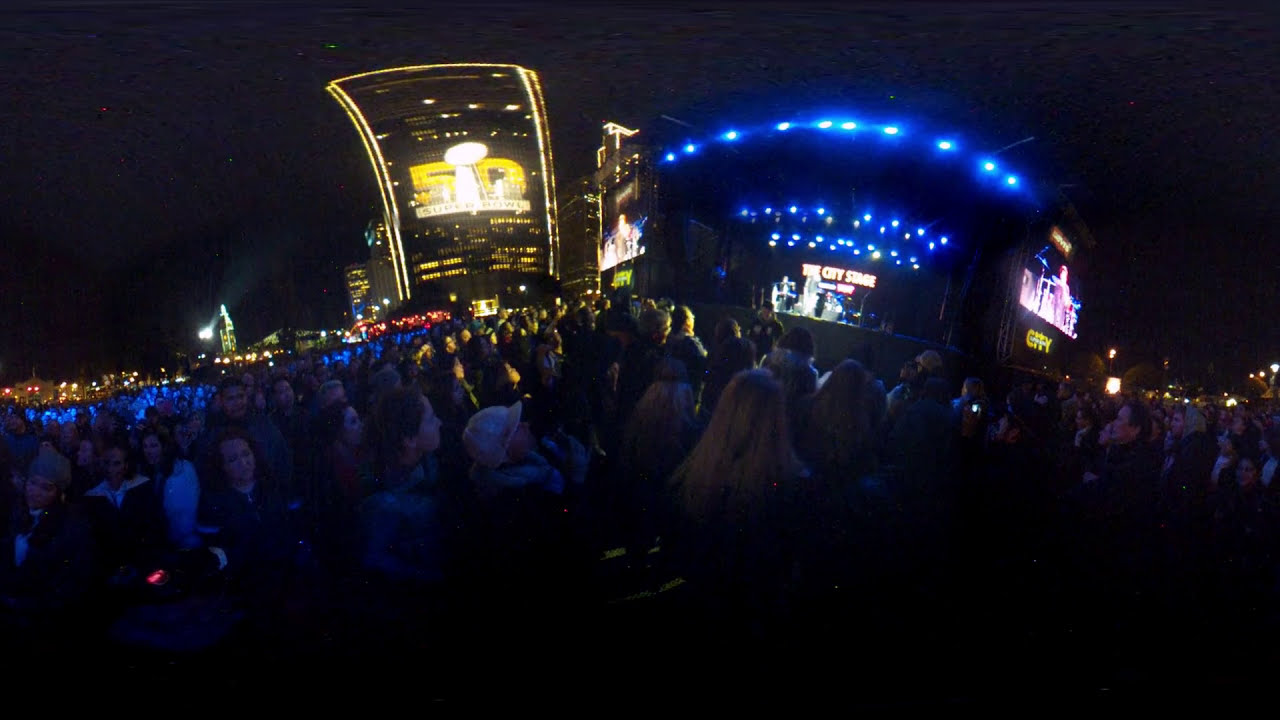The image depicts a vibrant night concert scene captured in a 360-degree photo. In the forefront is a large, densely packed crowd of people, facing a prominently illuminated stage that is slightly off to the right of the image's center. The stage is bathed in an array of colorful lights, including blue ceiling lights, and features the words "The City Stage" glowing in red neon at the back. 

Members of a band can be seen performing on stage, with additional stage lighting in different tiers enhancing the dramatic visual. To the far right, a tall building marked with bold, gold numeric characters "50" (possibly "5D" due to the visual distortion) stands out prominently. The concert takes place outdoors under a dark night sky, with more distant buildings vaguely visible in the background. There is no readable text other than the "The City Stage" and the numeric "50" sign, but the overall atmosphere suggests an energetic live music event under the night sky.